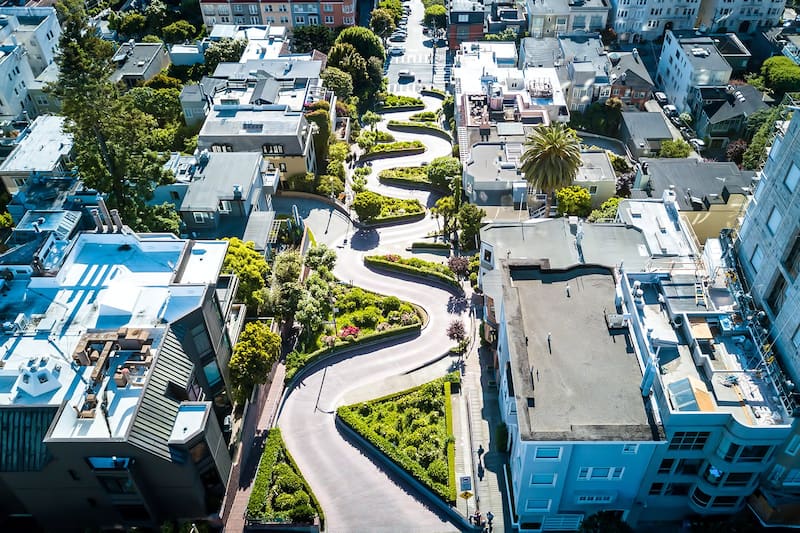This vibrant, full-color aerial photograph, framed with no borders, captures a sunny outdoor scene likely taken from a high vantage point in San Francisco. The central focus is the famously winding, serpentine road known as Lombard Street, distinguished as one of the crookedest streets in the world. This iconic, snake-like street winds through lush greenery with meticulously maintained topiary and shrubbery lining its sharp curves. Flanking the street are numerous substantial buildings, predominantly gray in color, varying from three to seven stories high, which could be residential apartments or commercial structures. The area appears affluent and well-developed, evidenced by the sophisticated landscape and the meticulously cared-for estates. A few parked cars are visible along the street, though no people can be discerned from this height. The scene extends to a bustling four-way intersection at the street's end, bordered by additional buildings. The bright daylight enhances the image's clarity, making every detail distinctly visible in this picturesque urban setting.